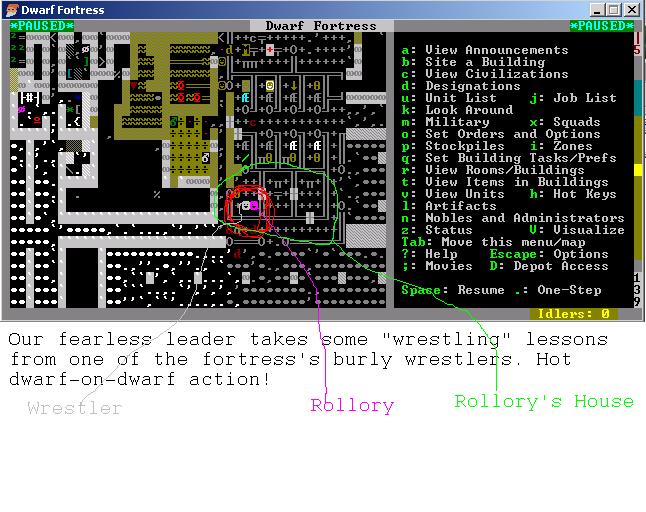This image is a computer game screenshot from the game "Dwarf Fortress." The screenshot displays a top-down view of the interior of a fortress, depicted with distinct rooms sketched out. The scene is primarily composed of black rooms bordered by gray lines, with notable features including a green room surrounded by white borders. The game interface includes a blue border at the top with the title "Dwarf Fortress," and below that, in green lettering, the word "paused." 

On the right side of the image is a panel that contains various game commands in white text, including options such as "View Announcements," "Site a Building," "View Civilizations," "Designations," and many more, approximately 20 options in total. 

Key areas in the fortress are annotated with colored text and pointers. For example, a red-circled section points to a character named "Rollery," identified in purple letters. Additionally, this annotation connects to a larger green-circled area labeled "Rollery's House" in green text. The annotations add context to the gameplay scene described below in black print, stating: "Our fearless leader takes some wrestling lessons from one of the fortress's burly wrestlers. Hot dwarf on dwarf action."

Overall, this detailed screenshot captures the intricate layout and interface of "Dwarf Fortress," highlighting specific characters, their locations, and essential game commands.